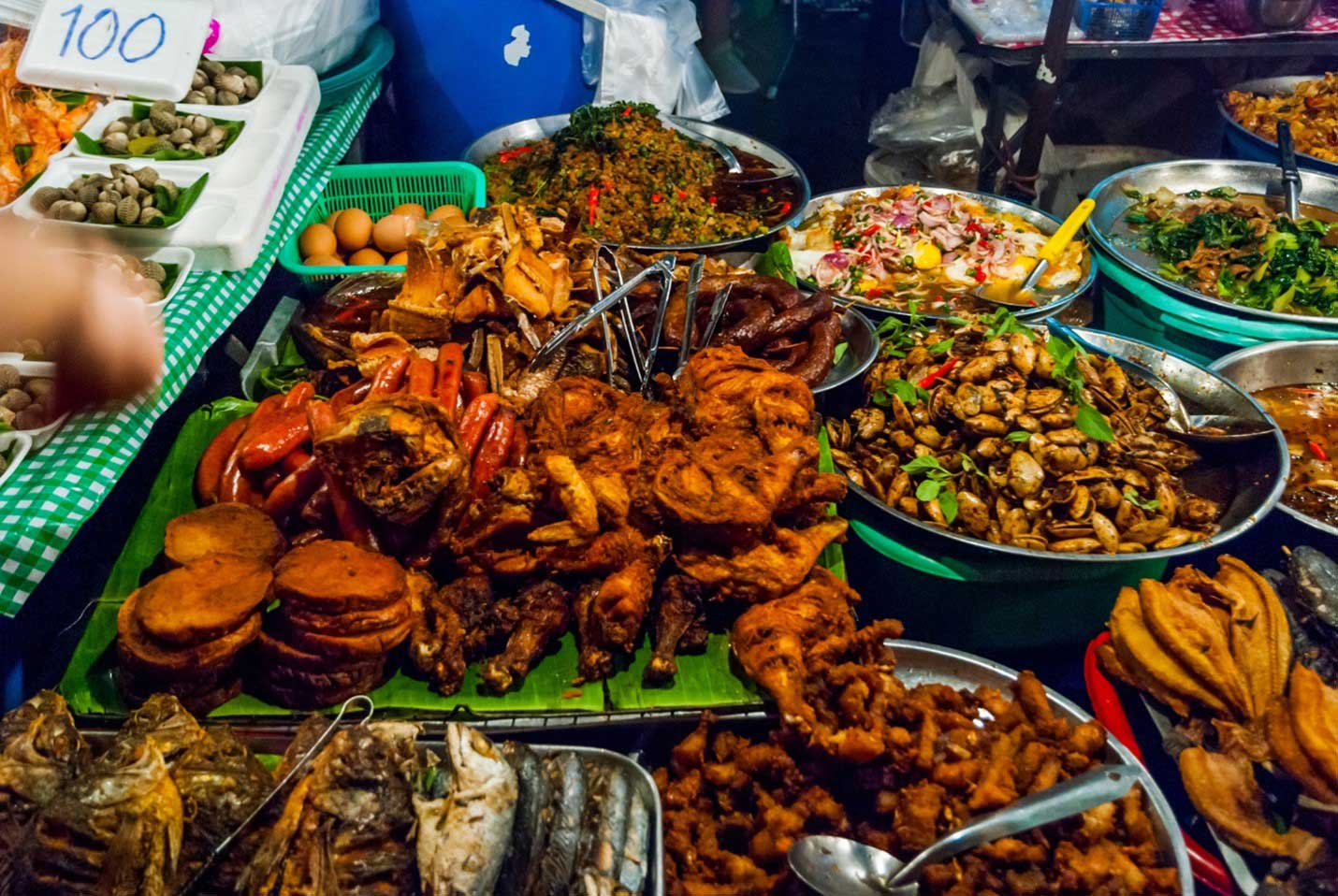The image captures an outdoor food vendor stall, possibly in an Asian market, with an array of dishes on display across multiple pans and trays. Central to the scene are various Asian cuisine elements, including roasted fish, fried chicken, and an assortment of seafood like crab legs and small shelled shellfish. Vegetables and rice dishes are also prominent, with broccoli-beef and vegetable-heavy varieties visible. A green bin holds brown eggs, indicative of balut or similar items. On the right, metal bowls contain broccoli and meat dishes, along with some fried foods possibly consisting of nuts or clams with green leaves. Fried patties and whole fish in a metal tray are situated at the bottom left, alongside another table with a checkered white and green tablecloth displaying additional dishes. The presence of a price tag with "100" written in blue, placed over individualized portions, suggests that customers pay for specific items, reinforcing the food vendor setting over that of a traditional buffet.